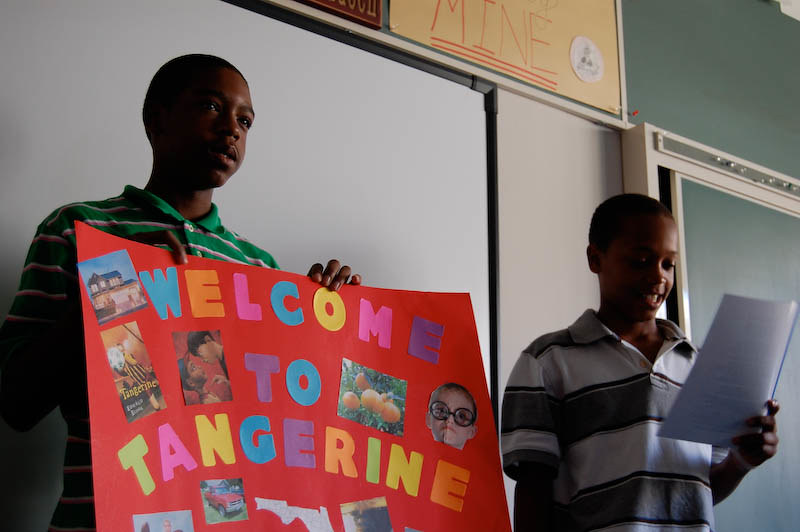In the image, two boys of color are standing in front of a classroom. Both boys are situated directly in the center of the image, with a whiteboard and a chalkboard visible behind them. The boy on the left, dressed in a green and white striped shirt, is holding up a red sign that says "Welcome to Tangerine." The sign is adorned with vibrant, multi-colored letters—each letter in a different hue such as blue, orange, pink, purple, and lime green—and features various pictures, including someone in glasses, tangerines, an illuminated house, and a map of Florida. To his right, the second boy, wearing a gray and white striped shirt, holds up a sheet of paper encased in a clear presentation folder with a bordered edge. Both boys appear to be engaged in delivering a presentation to their class, seemingly collaborating as a team. The setting suggests it is midday and likely within an educational environment.